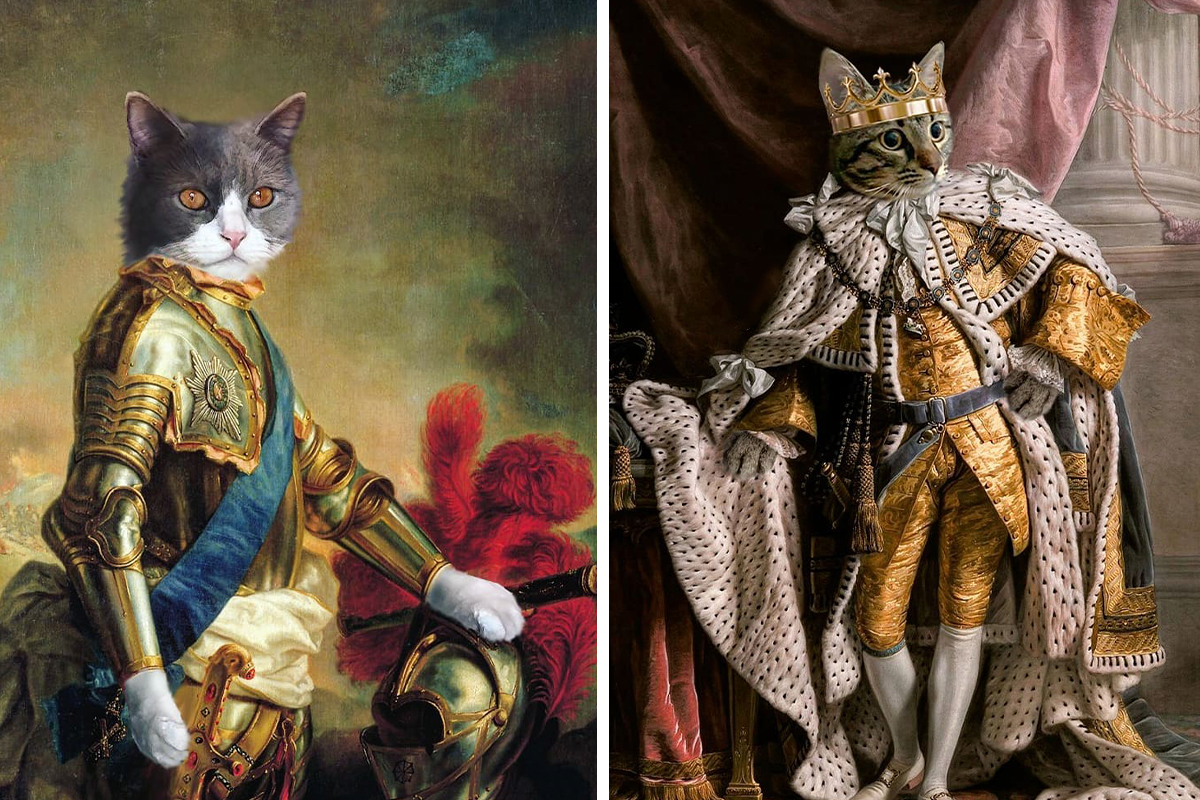The image is a composite of two separate portraits featuring cats dressed in extravagant, human-like attire from historical periods. On the left is a gray cat with a white snout and mouth, depicted in opulent, medieval-style gold armor. The armor is intricately detailed with silver and gold elements, and the cat's left paw, white and visible beyond the armor’s cuffs, rests on a helmet adorned with a striking red plume. 

On the right is a regal gray tabby cat, its head crowned with an ornate gold crown, signaling its royal status. The cat is dressed in elaborate, gold-lamelled clothing, including breeches, knee-length pants, white stockings, and a luxurious fur-trimmed white robe with black spots. The cat's right paw is elegantly placed on a table draped with a rich red cloth with dark brown tassels. Both portraits emphasize the cats' anthropomorphic representation, blending feline features with intricate Victorian and medieval human attire, showcasing a blend of whimsy and historical grandeur.